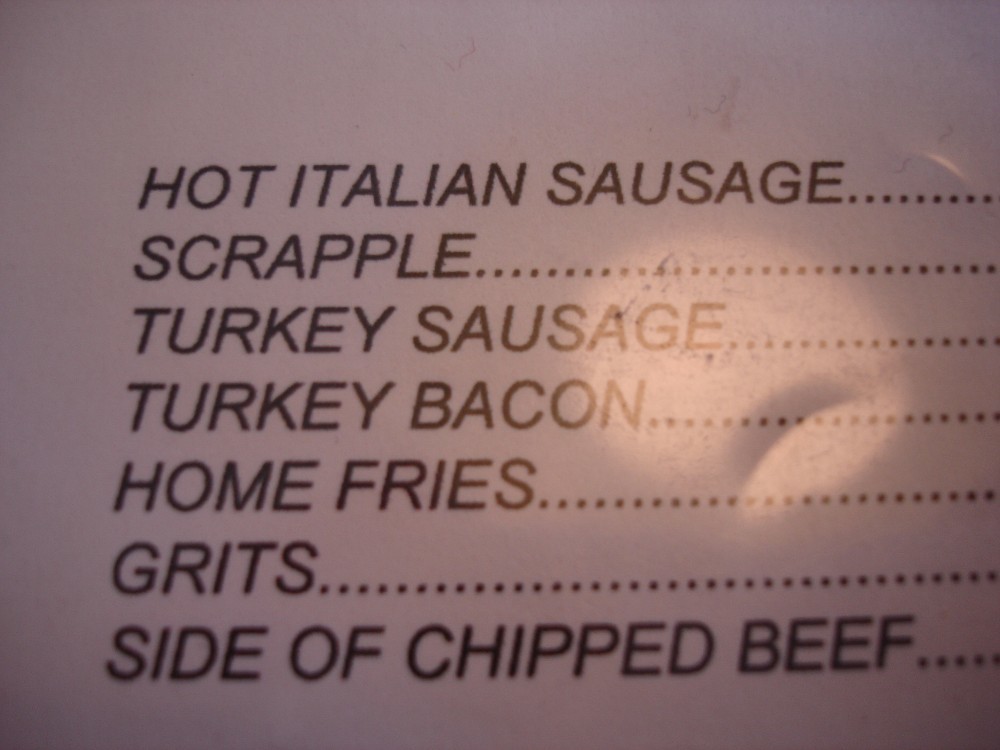The image captures a close-up shot of a menu, which is illuminated by a reflection of overhead lights situated towards the middle-right section. The first menu item listed is "Hot Italian Sausage," followed by "Scrapple," "Turkey Sausage," "Turkey Bacon," "Home Fries," and "Grits." The final menu item is "Side of Chipped Beef." Prices are not visible in this image; instead, a series of dots appear to the right of each food item. The menu's layout is straightforward, yet has a somewhat inventive design.